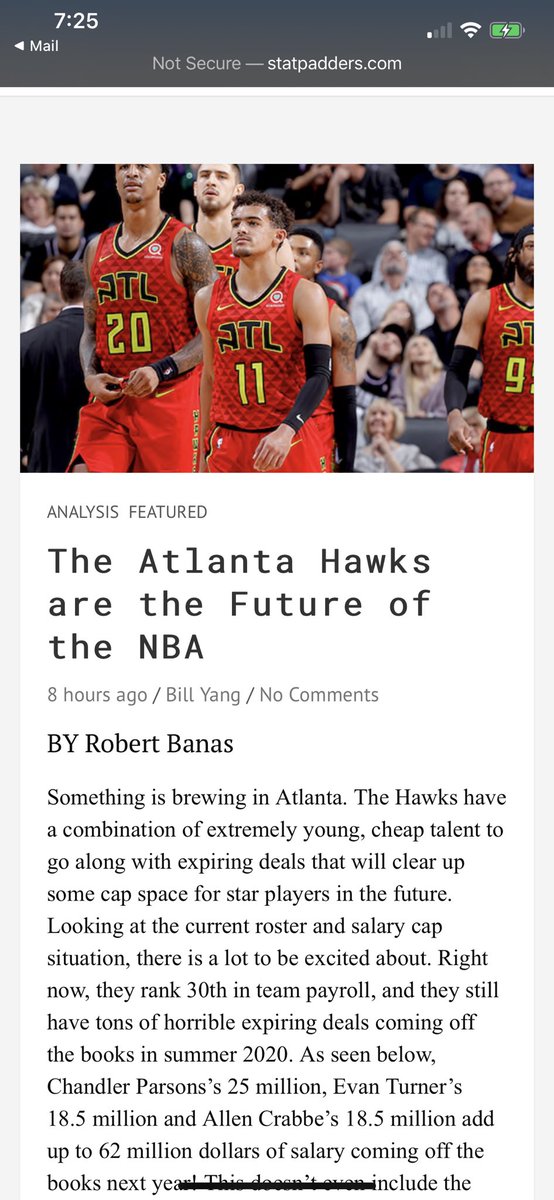This is a phone screenshot of an article discussing the Atlanta Hawks. At the top of the screen, the time reads 7:25, accompanied by the internet and battery charge icons. A small symbol pointing left is labeled "Mail." The URL at the top reads "notsecure-statpadders.com," indicating the site is not secure. Below the URL is an image featuring basketball players in red tank tops and red shorts with yellow numbers, emblazoned with "ATL" in black.

The main player in the foreground has a light tan complexion, curly black hair, and a goatee. To his left is a taller, light-skinned Black player with numerous tattoos on his arms. Behind these two, a White player with a goatee and short hair is partially visible. To the right, another player, possibly Hispanic, sports a long beard and has a glove on his arm. The background reveals a crowd of spectators, all looking upward, likely at a scoreboard.

The article, titled "Analysis Featured," is headlined "The Atlanta Hawks are the Future of the NBA." It was published eight hours ago by Bill Yang, with no comments, and authored by Robert Banas. The text begins by asserting that something promising is developing in Atlanta. It highlights the team's combination of young, affordable talent and expiring contracts that will soon free up substantial cap space. The article notes that the Hawks currently rank 30th in team payroll but have a significant amount of expiring deals that will clear by the summer of 2020, potentially freeing $65 million from contracts like Chandler Parsons' $25 million, Evan Turner's $18.5 million, and Allen Crabbe's $18.5 million. The article hints at more details but is cut off at this point.